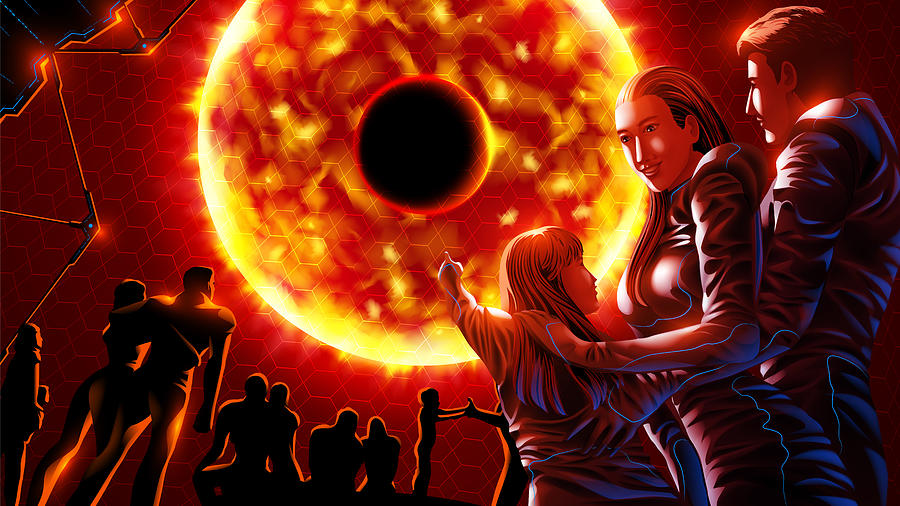This animated, digitally created image depicts a futuristic scene centered around a massive, fiery sun-like object with a darker red and orange, donut-shaped appearance. The central astronomical body features a black hole in its middle and is surrounded by intense flames radiating outward. The scene is set against a predominantly red backdrop with blue and orange hues and honeycomb patterns.

A crowd of shadowy silhouettes occupies the lower left corner, positioned in various stances—some sitting, some standing—all gazing up at the celestial event. Within this crowd, distinguishable are couples, including one pair standing close, and another individual facing and holding hands with someone else nearby.

On the right side of the image, a family stands distinctly visible in the midst of the scene. The family, dressed in futuristic jumpsuits adorned with light blue tiger-like stripes, comprises a man, a woman, and a young girl. The man stands at the far right, with the woman in front of him, her hand resting on the girl’s shoulder. The girl, visibly curious and engaged, points toward the spectacular, sun-like object, capturing the awe and wonder of the futuristic display they are witnessing together.